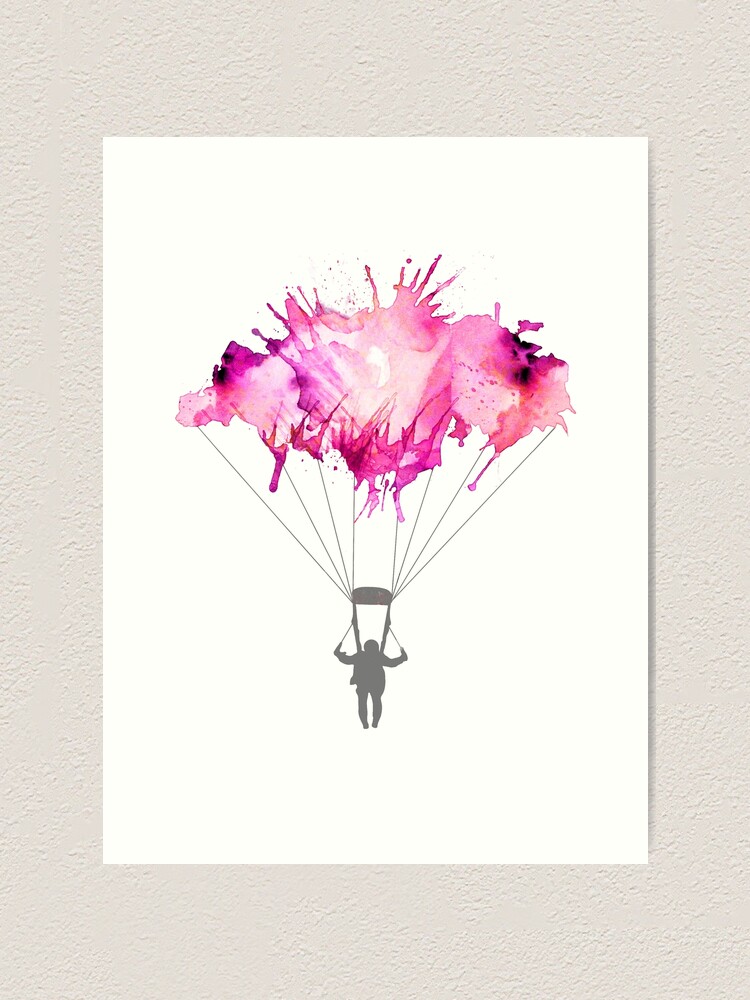This image captures a detailed painting mounted on a textured wall that is light gray with a rough surface. The painting itself is presented on a rectangular white background, slightly longer vertically than horizontally. At the base of the painting, there is a small gray silhouette of a person holding onto parachute strings. These strings stretch upward to connect to the parachute, which is depicted in an abstract manner. The parachute features a mix of pink, light pink, soft cream, and purple splotches, giving it a watercolor or inkblot appearance. The overall composition gives a sense of abstract elegance with a blend of textures and colors. A subtle shadow is cast on the right side of the white background, adding depth to the artwork.